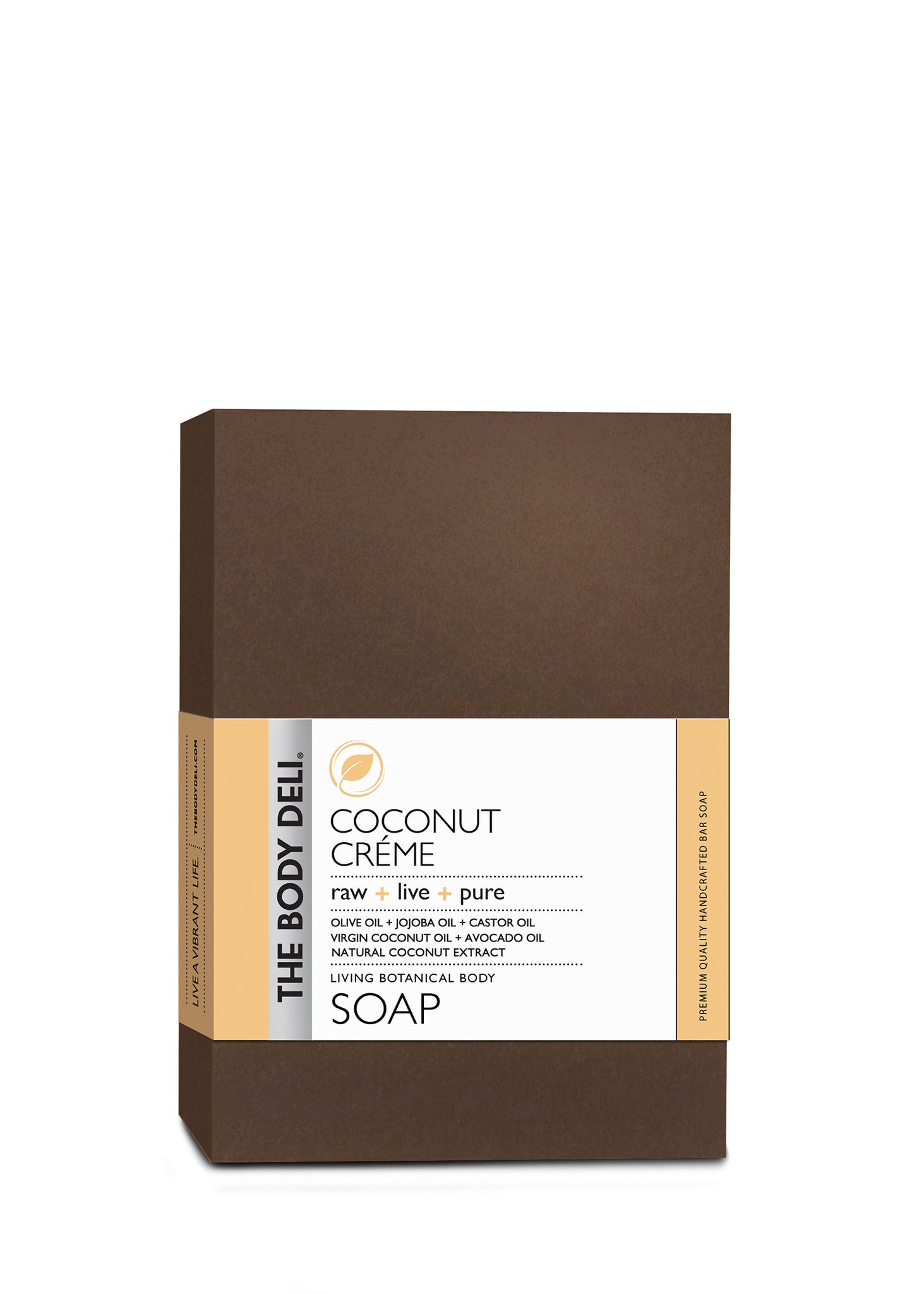The image depicts a rectangular-shaped bar of soap, appearing more like packaging or a digital representation rather than an actual bar. The primary color of the packaging is dark brown, accented with tan and white. The label, wrapped about three quarters of the way down, prominently features "The Body Deli" vertically and includes a decorative gold or tan leaf in the center. The label describes the soap as "Coconut Cream," emphasizing its raw, live, and pure ingredients, which include olive oil, jojoba oil, castor oil, virgin coconut oil, avocado oil, and natural coconut extract. The soap is identified as "Living Botanical Body Soap," highlighting its premium quality and handcrafted nature. The background of the image is plain, keeping the focus solely on the soap packaging.